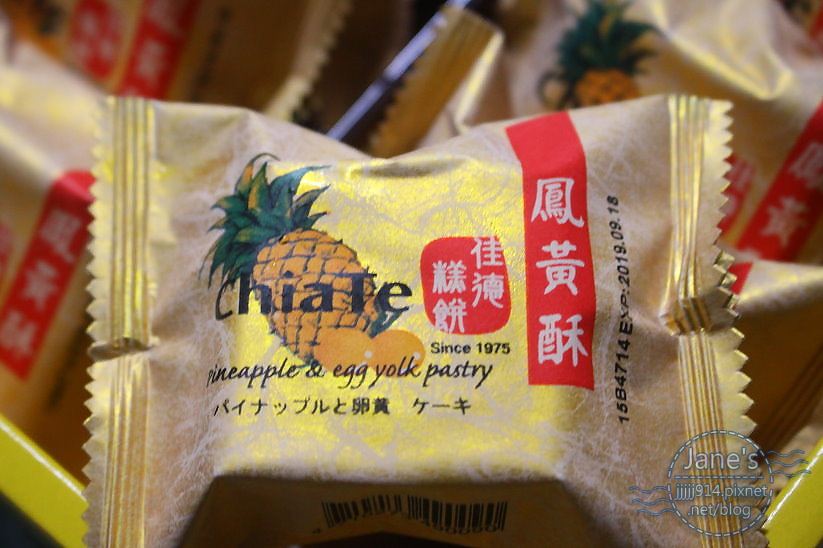The image depicts an up-close photograph of gold foil-wrapped pastries labeled as "pineapple and egg yolk pastry." The packaging features a predominant graphic of a pineapple and two egg yolks, with the brand name "Chia Te" (spelled C-H-I-A-T-E) positioned above the pineapple. In smaller English text below the graphic, it reads "pineapple and egg yolk pastry," and there is some Japanese or Chinese script present, particularly within a red rectangle on the right side of the wrapper. The packaging also notes the founding year with "Since 1975." The golden wrapper has a crinkled texture and jagged edges where it has been sealed. Additional details include an expiry date of "2019 09 18" and a barcode at the bottom of the wrapper. In the bottom right corner of the image, there is a watermark that reads "Janes JJ JJ J 9 1 4 pics.net/blog." Multiple similar pastries can be seen out of focus in the background, giving the impression of a collection of these treats.